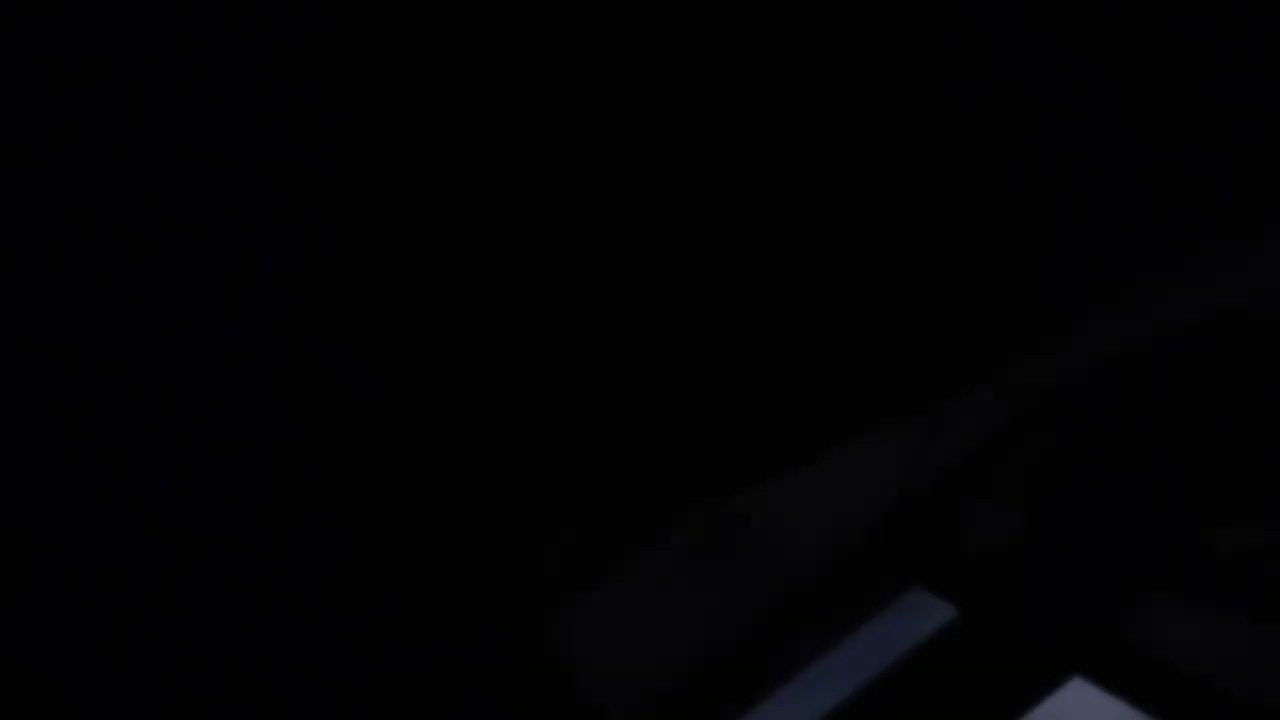The image features a nearly pitch-black background in a horizontal rectangular shape, with only a faintly visible gray object peeking out from the bottom-right edge. This object, possibly resembling a corner of a striped blanket or towel, includes a light gray stripe at the top, followed by a black stripe, and a gray triangle pointing upward with its base parallel to the bottom edge. Both the gray object and the gray stripe are angled obliquely. The image's predominant darkness gives the impression of an inadequately lit scene, perhaps illuminated by a distant streetlight, making the true nature of the gray elements difficult to discern.